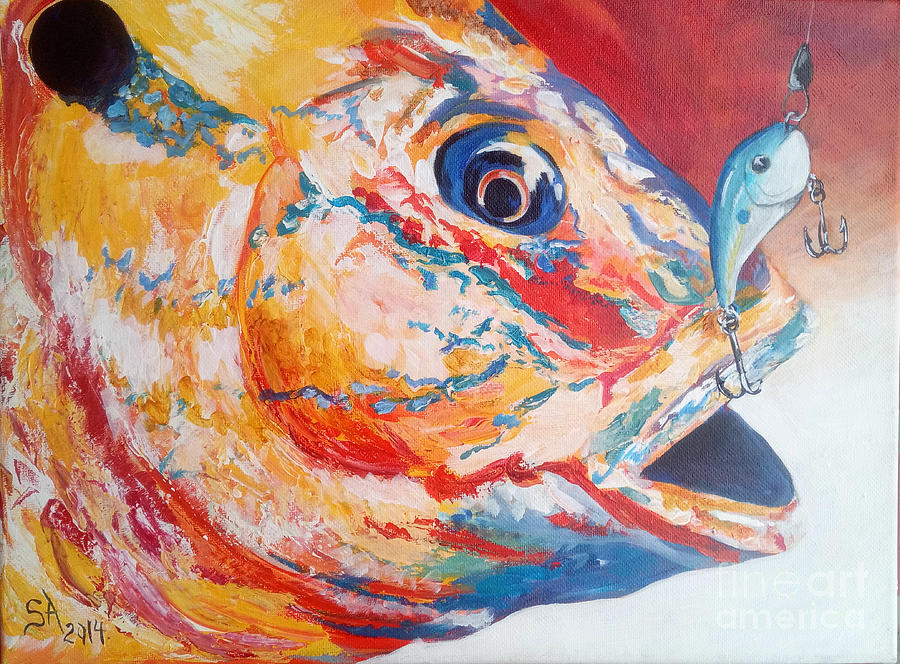This is an oil painting capturing a close-up profile of a multicolored fish with red, white, blue, orange, and yellow splotches. The fish, swimming towards the right, has its mouth open, revealing a silver hook embedded in its top lip. Attached to the hook is a smaller, blue fish lure with another hook protruding from its body. The large fish’s eye and textured scales demonstrate intricate detailing. Visible brush strokes and canvas texture add depth to the piece. The background features a gradient from red at the top to white at the bottom. In the bottom left corner, the text "SA 2014" is written in black, while the bottom right corner showcases a transparent watermark reading "Fine Art America."